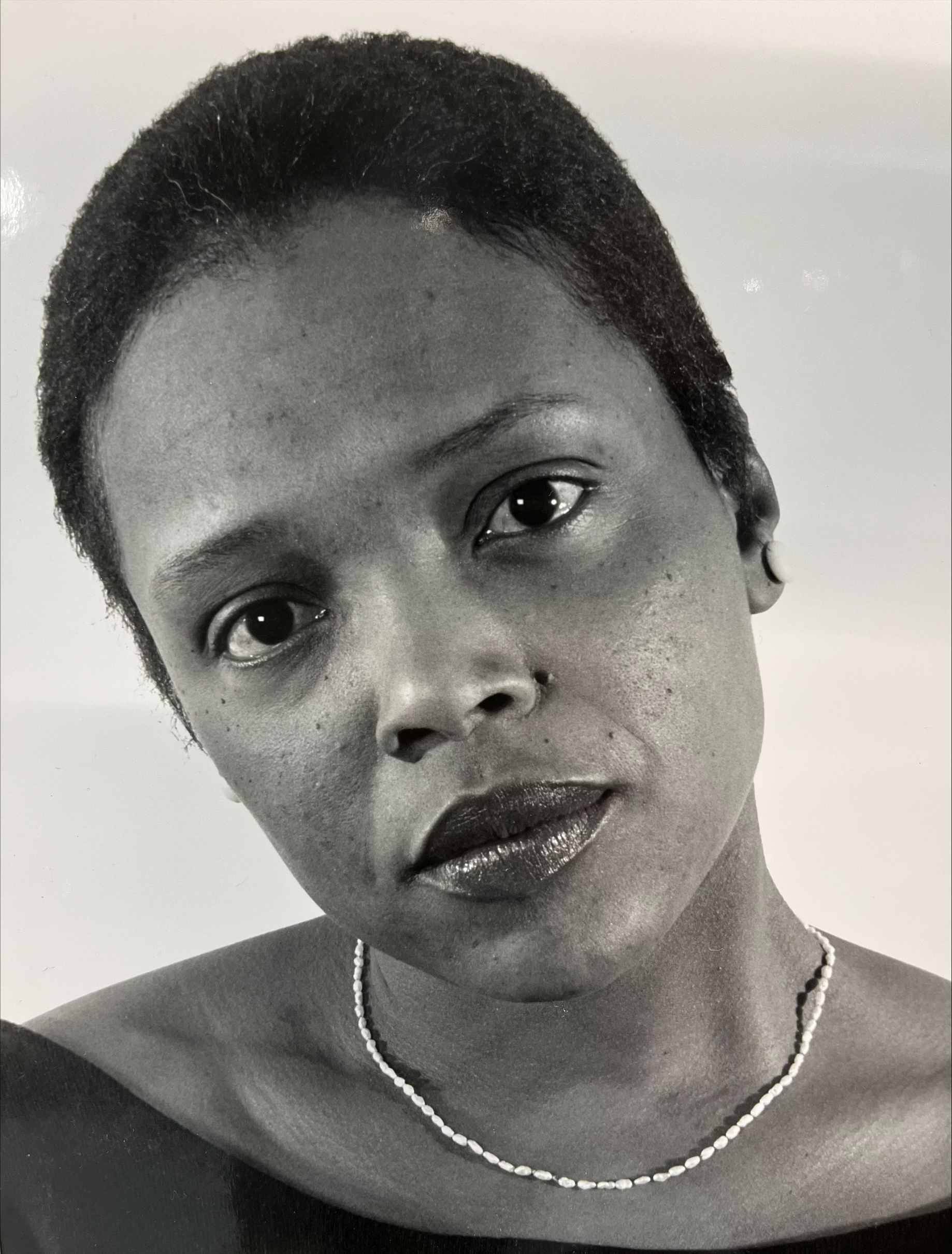This close-up image captures a young African American woman named Eva Golson. She has short, black hair and her head is slightly tilted to the side as she gazes curiously into the camera. Eva's expression resembles the quizzical look one might give while watching children and thinking, "What are you up to?" She wears a subtle touch of red lipstick on her lips, and her dark eyebrows frame her deep, dark eyes. Her nose, wide at the base, adds to her distinctive facial features, complemented by a small mole to the right of it. Eva is adorned with a small, white beaded necklace around her neck and her attire includes a black top that gently rests on her shoulders. Her ears are accessorized with white flat button earrings. The photograph has a minimalist background in a grayish cream color with specks of white, ensuring that Eva's striking features remain the focal point. Despite a few zits on her cheeks, the portrait radiates her natural beauty and contemplative demeanor.